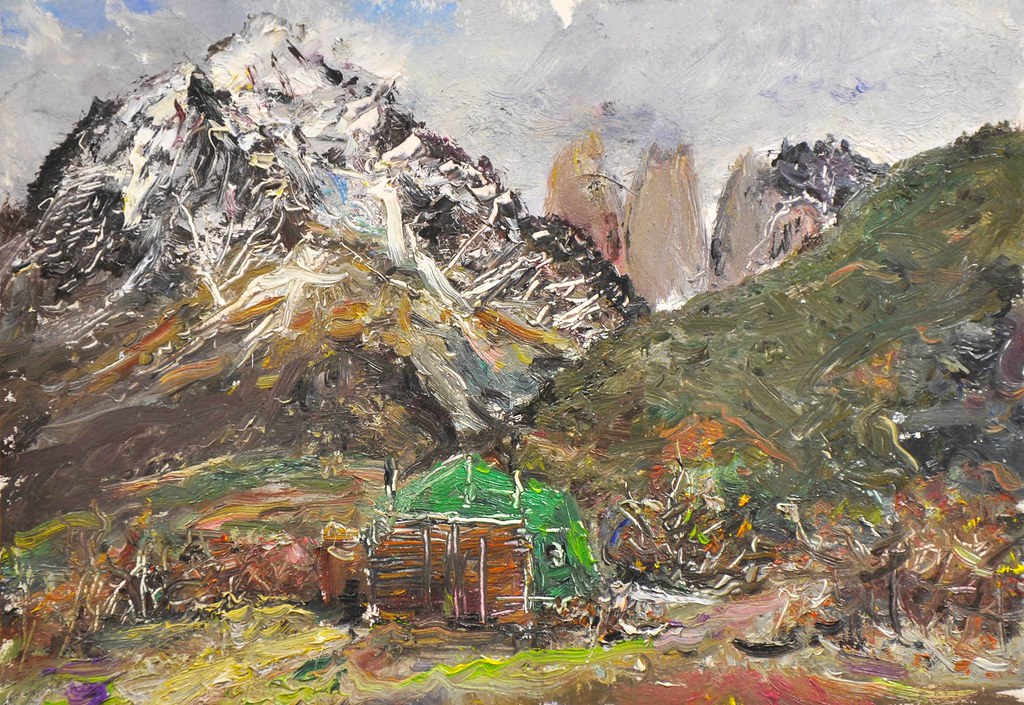This painting, rendered in an Impressionist style, depicts a mountainous landscape with a small green shack, possibly made of wood, sitting at the base. The artwork showcases a couple of mountains, one of which is prominently covered in a blend of brown, black, and abundant white strokes suggestive of snow, standing tall against a cyan sky where gray clouds are forming. The other mountain range, located closer to the foreground, is enveloped in green hues, indicating lush grass with interspersed touches of brown and gray. Overall, the colors employed are a mixture of earth tones—bright green, evergreen, brown, auburn, red, and flecks of yellow—applied in a non-uniform, splattered manner. The scene is set during the day, with the abstract, broad brush strokes clearly visible, contributing to the painting’s dynamic yet cohesive depiction of nature.